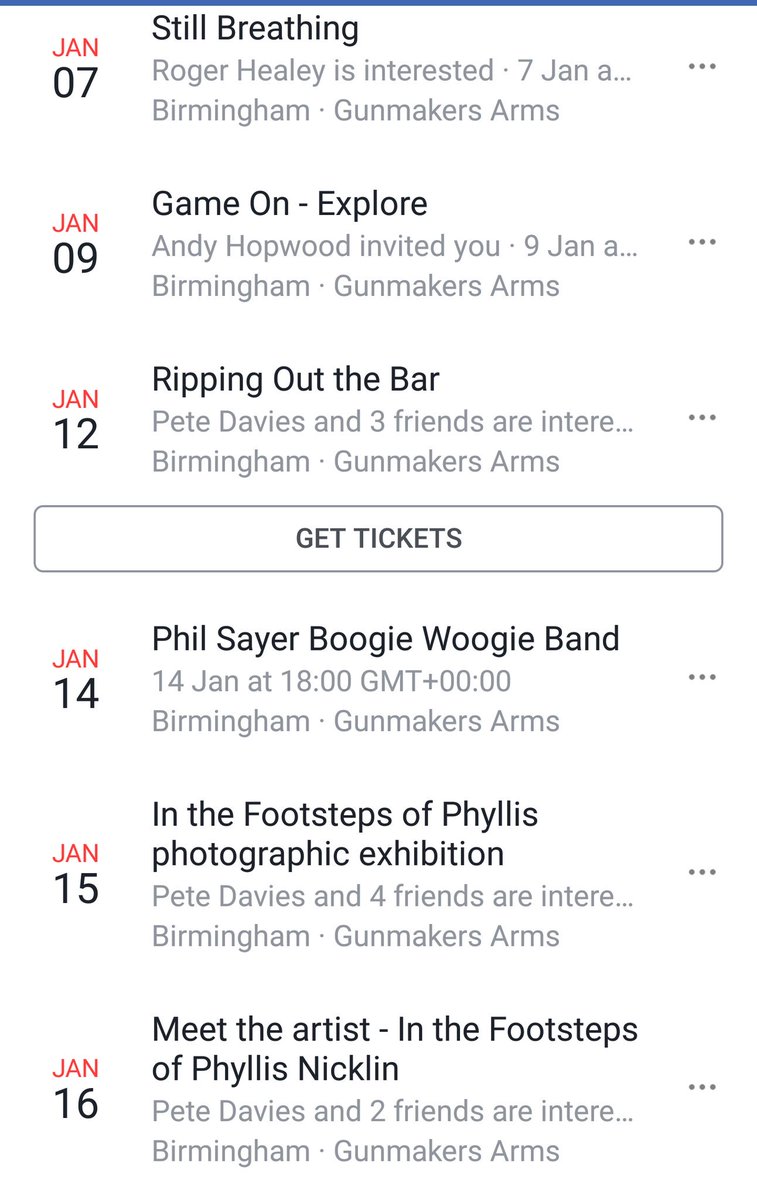**Descriptive Caption:**

A detailed screenshot from a smartphone display features a notable blue line spanning from left to right at the top of the screen. Below this line, the words "Still Breathing" are prominently displayed in black, with capitalized letters 'S' and 'B'. To the left of this text, the all-caps abbreviation "JAN" (January) followed by "07" in a black font. Adjacent to these, in gray, appears "Roger Healy is interested" next to the number "7", followed by "JAN" in uppercase and "a..." in lowercase with three gray dots trailing this text. Three dark dots are positioned to the far right.

Below this section, the text "JAN 09" is displayed, followed by "Game On - Explore" with capitalized initial letters. Lower down, "Andy Hopwood invited you" is in gray, followed by "9 JAN" with a capital 'J' and lowercase 'a' trailed by three gray dots and three darker dots to the right.

Further down, "JAN 12" appears in all caps, followed by "Ripping out bar" with capitalized 'R', 'O', and 'B'. Below this, "Pete Davies and three friends are interested", with the initials 'P' and 'D' in uppercase, trailed by "inte..." and ending with three larger gray dots alongside three dark dots.

The text "Birmingham. Gun Makers Arms." is positioned above a gray rectangular box centered with the text "GET TICKETS" in dark letters and all caps.

The text "JAN 14" is next, accompanying "Phil SWB Band" to the right, followed below by the date "14 JAN at 18:00 GMT +00:00" in gray, with three dots to the right. Beneath this, "Birmingham. Gun Makers Arms." is reiterated, followed by "JAN 15" in red lettering.

Next, "The Footsteps of Phyllis" is displayed, leading into the "Photographic Exhibition" with "Pete Davies and four friends are interested". 

Finally, "JAN 16" in black, followed by "MEET the artist - In the Footsteps of Phyllis Nicklin" with capitalized initials "I" and "F" in both titles, and gray text "Pete Davies and two friends are interested", ending with a recurrence of "Birmingham. Gun Makers Arms.", each text section trailed by three gray dots, and distinct patterns of three gray and darker dots.